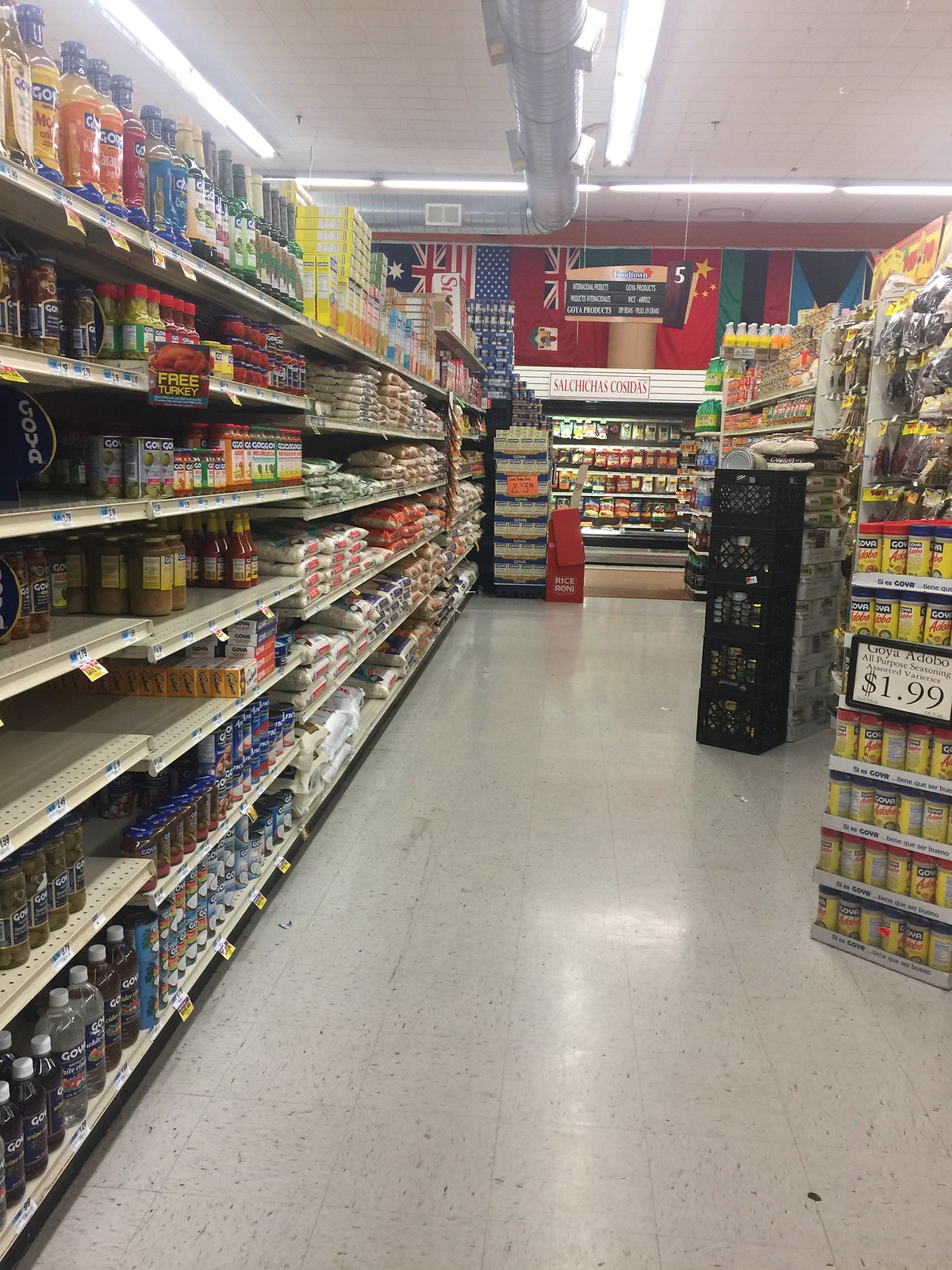In the photograph, we find ourselves inside a bustling grocery store, characterized by its white, speckled commercial floor tiles. The scene is filled with vibrant racks and shelves stocked with a diverse range of food items. To the left, the shelves are brimming with various sauces, alongside neatly stacked bags of rice and beans, showcasing a rich assortment of staple foods. On the right, there are numerous bags filled with dried herbs, adding an aromatic element to the visual. In the distance, a refrigerated section is visible, featuring an array of hanging products, likely perishables. The signage throughout the store hints at it being located in a Spanish-speaking country, as none of the signs appear to be in English.